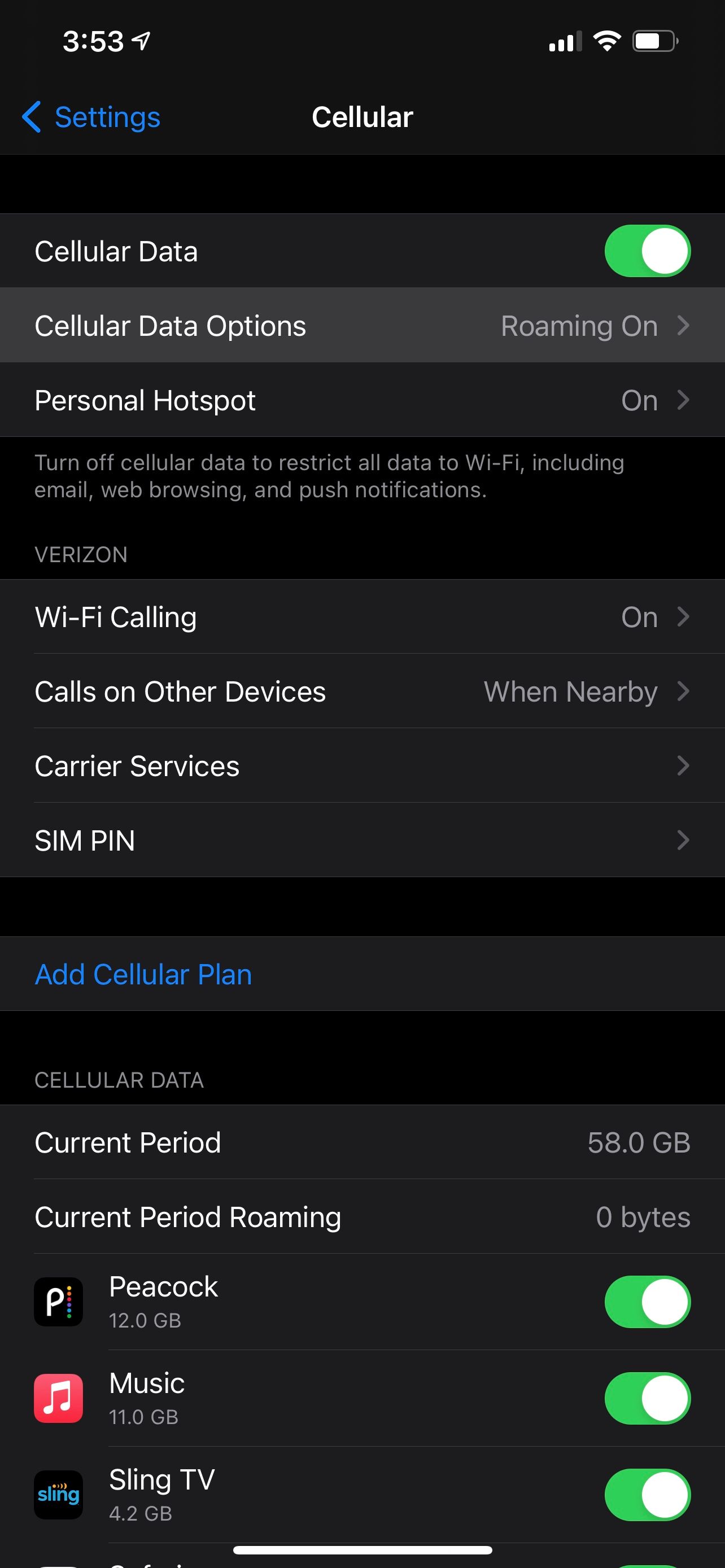The screen capture showcases a detailed view of a cell phone screen using a dark theme with a black background. 

At the top left corner, the status bar displays "3:53" in white text with an upward-right arrow. On the upper right, the status icons include three white Wi-Fi bars, the Wi-Fi signal symbol, and the battery icon.

Below the status bar, centrally aligned in white text, it reads "Cellular." On the left, in dark blue text, it says "Settings" accompanied by a back arrow also in blue. 

The subsequent lines feature white text detailing various settings:
- "Cellular Data" with a green toggle switch indicating it is currently turned on.
- "Cellular Data Options" with a note stating that roaming is on.
- "Personal Hotspot" which is also enabled.

Underneath these settings, a message advises: "Turn off cellular data to restrict all data to Wi-Fi, including email, web browsing, and push notifications."

Further down on the left, the user's carrier information is displayed in white:
- "Verizon" (the carrier)
- "Wi-Fi Calling" is enabled.
- "Calls on Other Devices" when nearby.
- "Carrier Services"
- "SIM PIN"

A blue header labeled "Add Cellular Plan" appears next, followed by more settings in white text:
- "Cellular Data" usage details show:
  - "Current Period: 58 GB"
  - "Current Period Roaming: 0 Bytes"

Lastly, there are three app icons:
1. To the left, the "Peacock" icon with "Peacock" text to the right.
2. An orange square with a music note and "Music" text to the right.
3. The "Sling TV" logo with "Sling TV" text to the right.

Each of these app entries has a green toggle button, all of which are turned on.